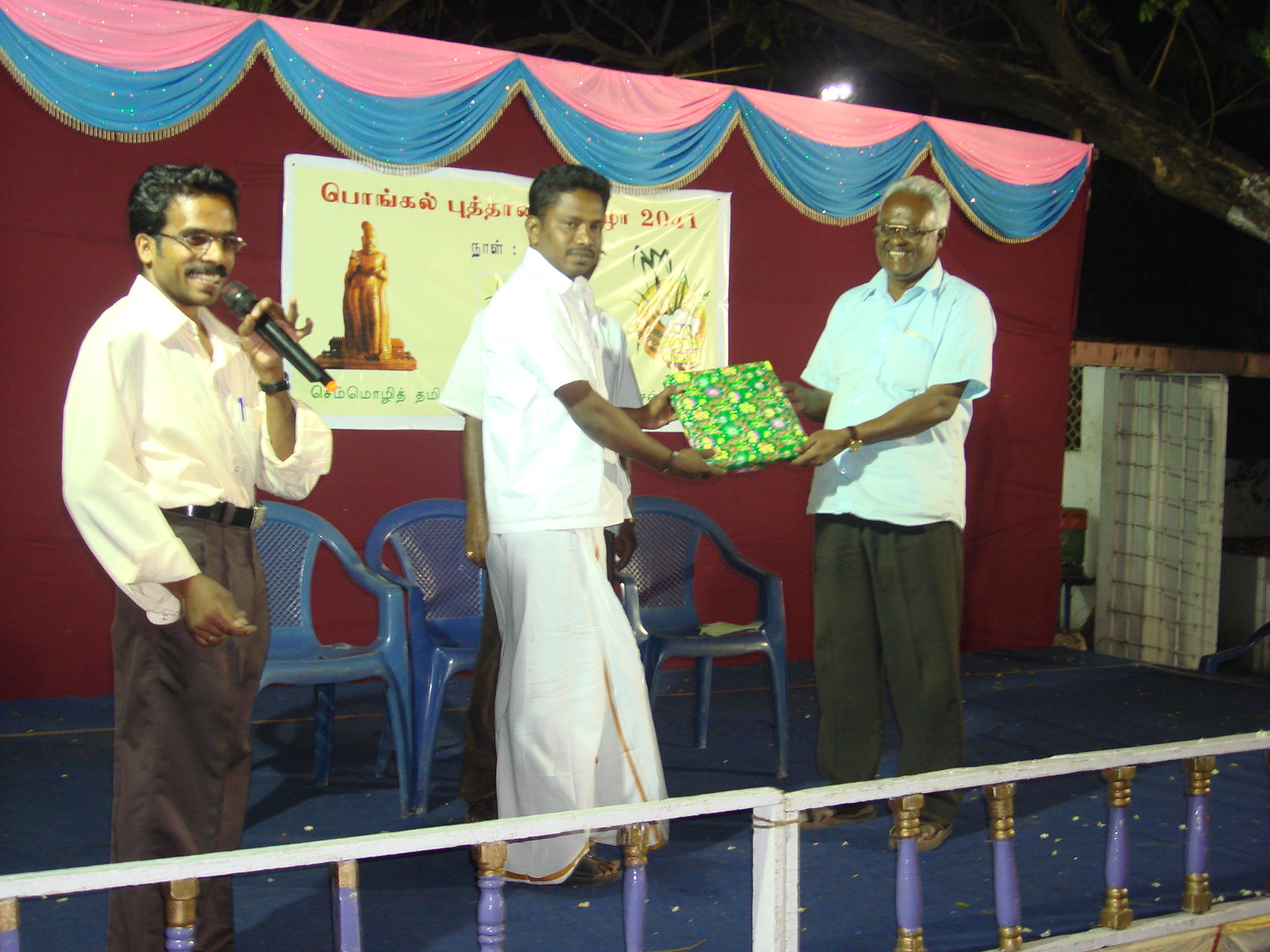In this vibrant image, three men of likely Indian descent stand on a stage adorned with a blue floor and a colorful backdrop of red, blue, and pink curtains. The man on the left, dressed in light-colored clothing and brown pants with a black belt, is in mid-speech, holding a microphone to his mouth. The central figure, wearing white bottoms, and the third man, also with a light-colored shirt, black trousers, and brown shoes, are prominently displayed holding what appears to be a gift wrapped in green floral wrapping paper, possibly indicating a celebratory occasion. Their smiles suggest a joyful moment, further amplified by the intricate backdrop featuring Indian text and a golden statue. Behind the men are three blue plastic chairs, hinting they recently rose to present or accept the gift. A barely visible fourth man is partially hidden but positioned close to the group, contributing to the convivial atmosphere.